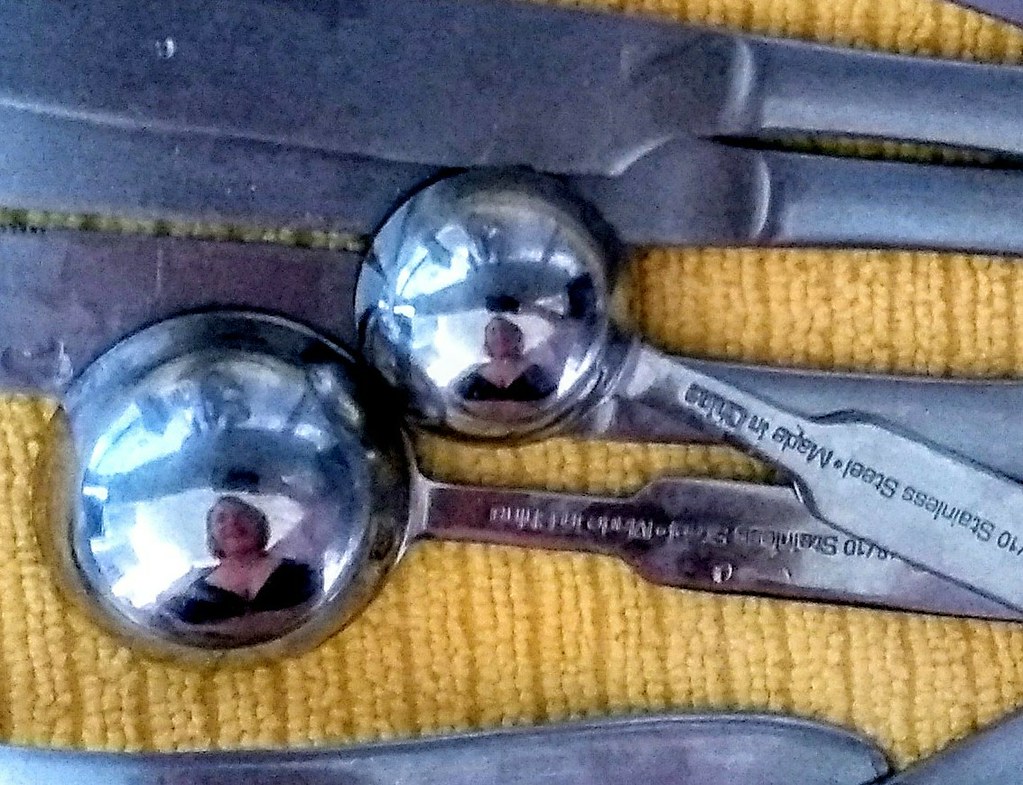This highly detailed up-close photograph showcases various pieces of silverware meticulously arranged on a yellow kitchen towel. Prominent in the center-left of the image are two upside-down measuring spoons, one resembling a teaspoon and the other a tablespoon, clearly marked with text that ends with "stainless steel made in China." Both utensils reflect the image of a woman, likely the photographer, who has short hair and is wearing a black shirt. Above the measuring spoons, three butter knives lie horizontally with their blue-gray handles and darker gray blades contrasting against the gold towel. Finally, at the bottom of the photo, the curved gray handle of another piece of silverware, though incomplete, adds to the composition of this vibrant yet intimate snapshot.